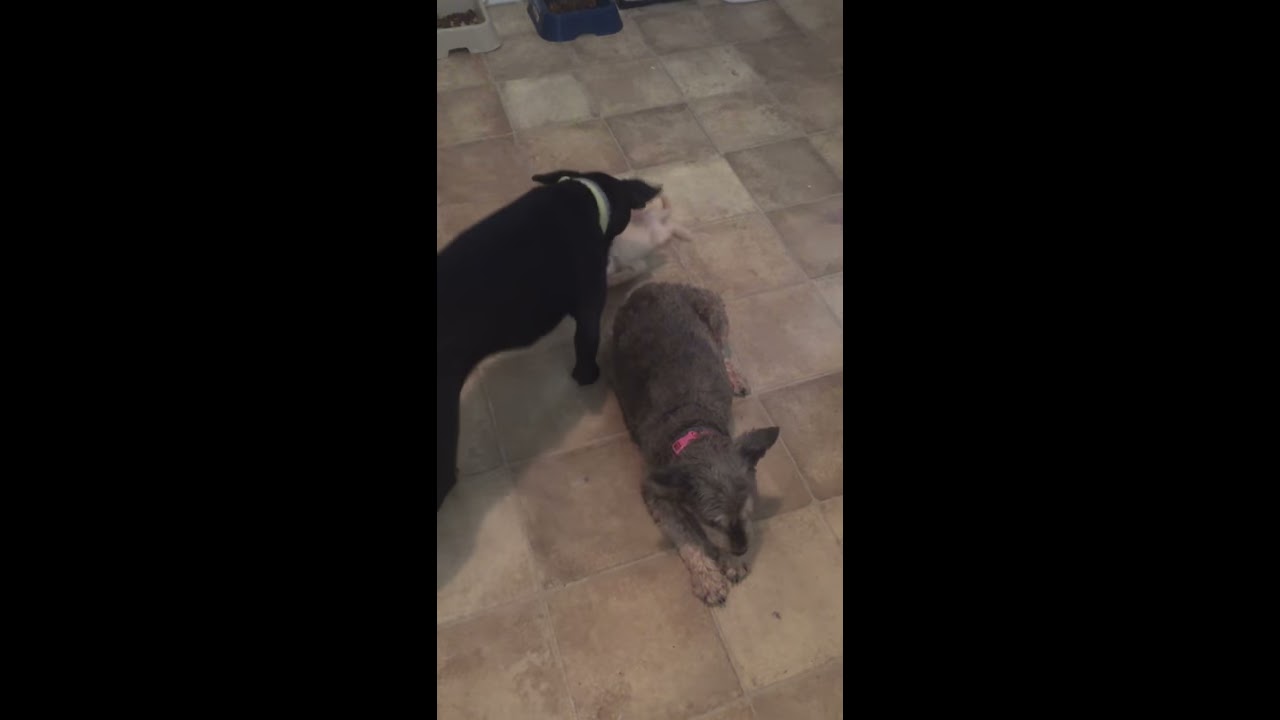This detailed portrait photograph captures three dogs in an indoor setting, all positioned on a light brown, tiled floor with varying shades of beige and tan. Dominating the scene, a black dog, sporting a neon green collar, stands on the left, its back turned to the camera, obscuring its face. Adjacent to it, closer to the center, a gray dog sits calmly, adorned with a pink collar that could be a bow. This dog's lighter gray paws contrast with its darker gray body. To the right, a smaller, light cream-colored dog lies on the floor, stretching its legs forward in a relaxed posture. In the top corner of the image, white and dark blue food bowls are conspicuously placed, hinting at the dogs' feeding area. The photograph's frame is vertically bordered by distinct black strips on both sides, enhancing the indoor setting's cohesive layout.